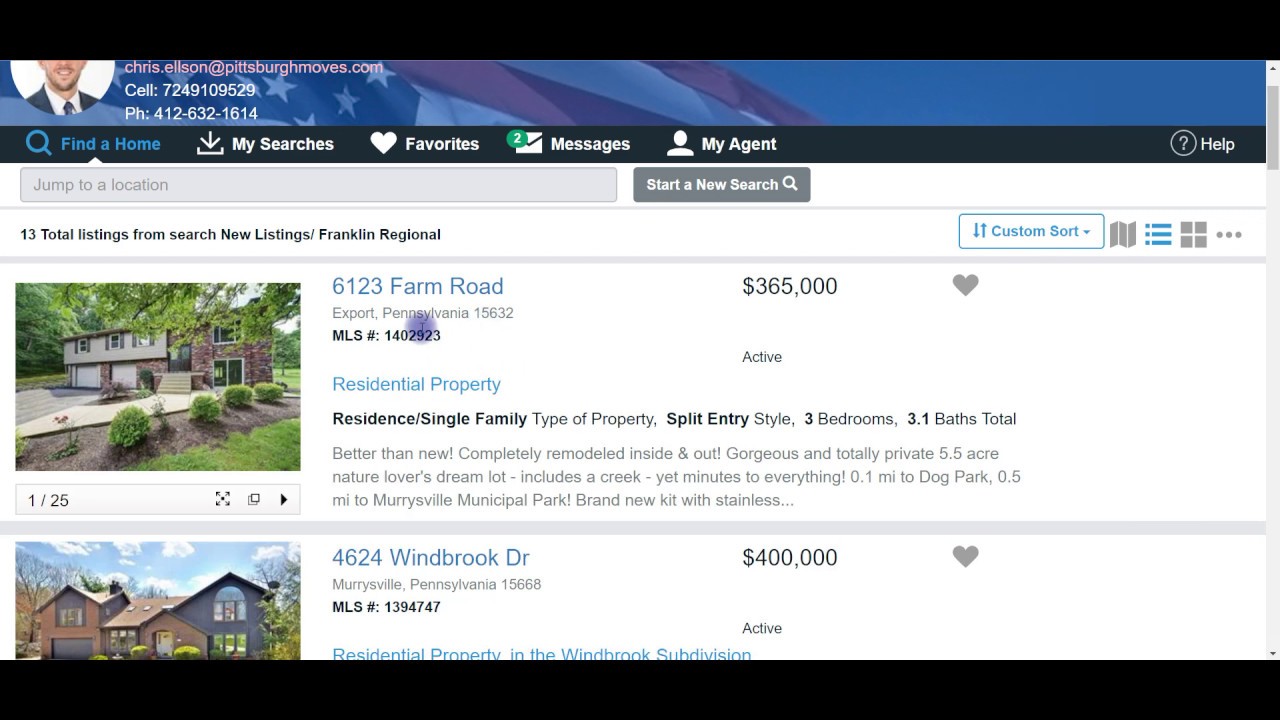The image features a black border at both the top and bottom. Below the top border, there is a cropped picture of a white man, partially obscured, wearing a black suit and a black tie. The background of his photo displays an American flag with a blue tint, making the entire upper section appear blue.

Next to the image, in pink text, the name "Chris Ellison" is displayed alongside a URL "PittsburghMovies.com" or "PittsburghMoves.com." Below this, in white text, is Chris Ellison's cell phone number: "724-910-9529," followed by his office phone number: "PH: 412-632-1614."

Underneath is a thin black border, and to its left, a blue magnifying glass icon labeled "Find a Home." On the right side are additional icons: a download icon labeled "My Searches," a heart icon labeled "My Favorite," and an envelope with a green circle and the number "2" indicating "Messages." Finally, there is a text that says "My Agent."